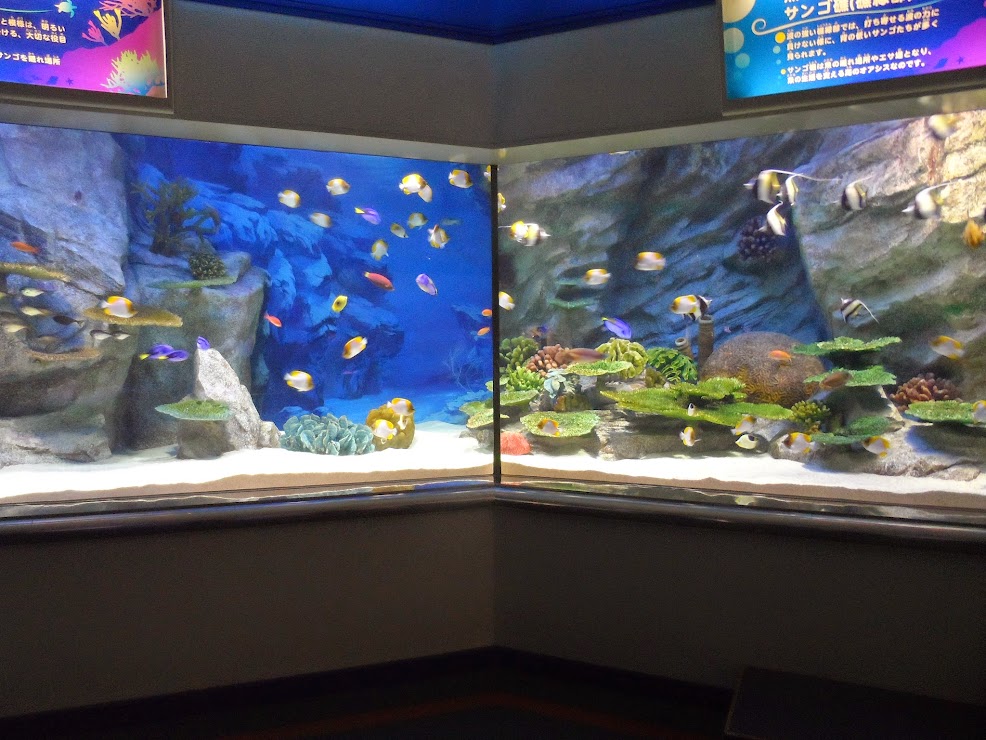The image depicts a section of an aquarium with two adjoining panels forming a corner, marked by murky quality suggestive of a photograph with a watercolor filter applied. The scene includes various brightly colored fish swimming amidst live coral and rock formations. The black floor and low grey wall give way to the aquarium panels, which display fish in hues of red, blue, yellow, white, and with distinctive stripes. Above the panels, Japanese signage hangs, with each corner of the aquarium framed by non-English text on the vibrant blue and magenta background. The absence of people emphasizes the serene aquatic environment.